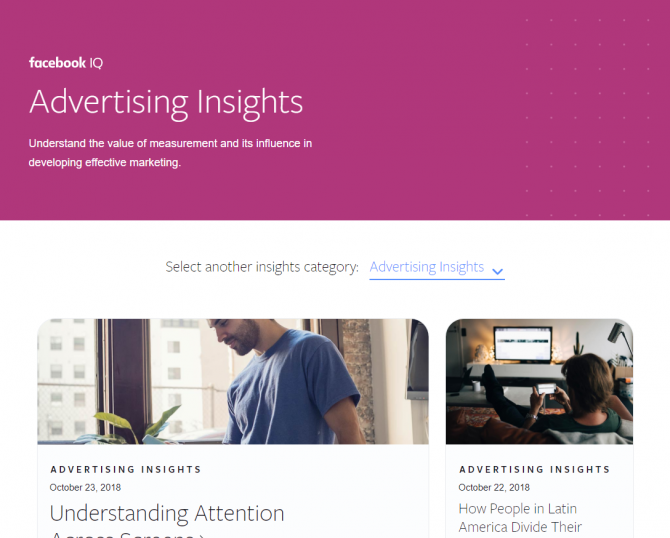This screenshot captures the Advertising Insights page from Facebook IQ, featuring a magenta header with white text. The header prominently displays "Facebook IQ" in small lettering at the top, followed by the main title "Advertising Insights" in large lettering. Beneath this, there is a subheading in very small lettering that reads, "Understand the Value of Measurement and its Influence in Developing Effective Marketing."

Below the header, the content is divided into two sections. The left section showcases an image of a man looking down at a planet, accompanied by a blog post titled "Understanding Attention," which was published on October 23, 2018. The right section features a photo of a man lounging with his feet up on a desk, playing a game with a computer in the background. This section is partially cut off but starts with the title "How People in Latin America Divide Their..." and the post date of October 22, 2018.